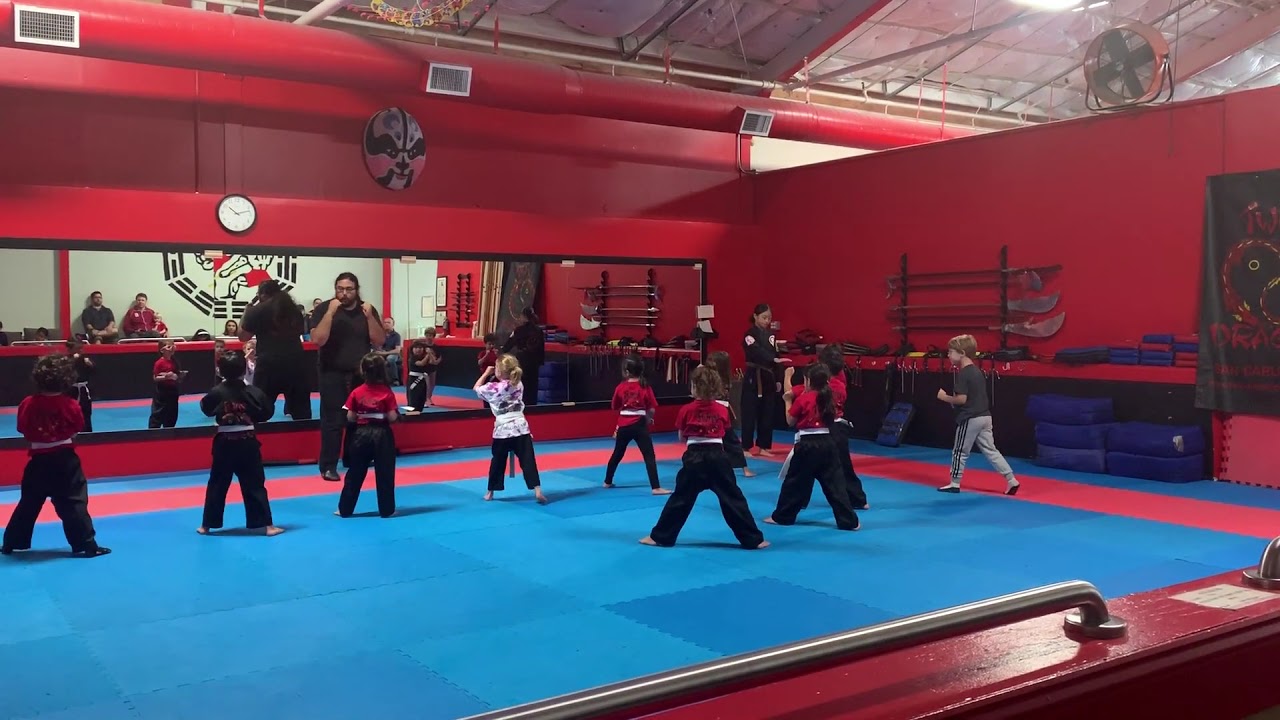The image shows the interior of a well-organized and clean martial arts dojo, possibly set up within a larger gym as the walls do not reach the ceiling. The dojo features red walls and soft, rubbery, blue floor tiles often found in children's play areas. At the center of the scene, a large man, the master, dressed in a dark shirt and pants with his hands up in a fighting stance, faces several children who are training in front of him. The children, spaced evenly apart, mostly wear red tops and black bottoms, with white belts around their waists, although some wear variations with white or black tops. Behind the instructor, a large mirror reflects the scene, including some adults observing from the back. A wall clock and a black-and-white martial arts mask are also visible, adding to the dojo's traditional decor. The blue mat beneath the students features a red stripe, enhancing the dojo's distinct color scheme.